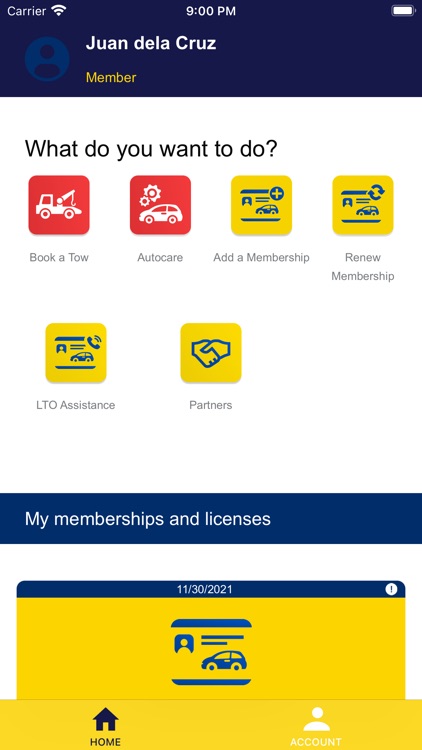The image depicts a mobile phone mock-up of a user's profile page with a blue, yellow, and white color scheme. In the upper left-hand corner, the status bar displays the text "Carrier" next to the Wi-Fi signal icon, with the time showing 9:00 PM and a full battery icon. The main profile area features a circular avatar displaying a head-and-shoulders illustration of a person. Below this, the name "Juan de la Cruz" is shown in white text, while the label "Member" appears in yellow text beneath it.

Immediately below the profile information, there is a white input field asking, "What do you want to do?". Across this field are four square icons: the two on the left are red with white icons, labeled "Book of Toe" and "Auto Care," and the two on the right are yellow with blue icons, labeled "Add a Membership" and "Renew Membership." Further down, additional options are displayed in yellow squares with blue icons, labeled "LTO Assistants" and "Partners."

A horizontal blue line divides the screen, with the text "My Membership and License" above it. Below this line, a yellow pop-up section extends from the bottom bar. This section, accented with a blue title, displays the date "11-30-2021" and an icon of a speeding car next to a driver's license image.

Finally, at the bottom of the screen is a yellow navigation bar featuring two sections. The "Home" section is marked in dark blue with a house icon, while the "Account" section is labeled in white with a simple person icon.